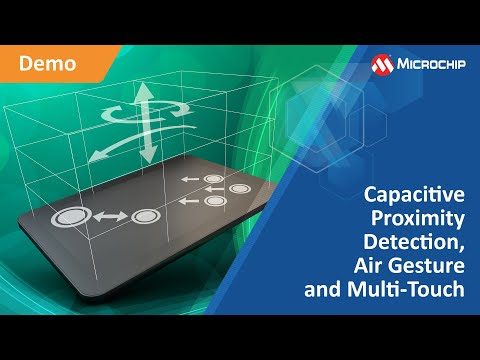The image is a detailed thumbnail promoting a product demonstration for a microchip, potentially part of a YouTube video or PowerPoint presentation. Dominating the upper right corner is the company's logo, a red circle with a white "M" inside, accompanied by the word "microchip." The image is framed by solid black stripes above and below.

In the top left corner, there is an orange text box labeled "Demo" in white letters. Centrally, the image showcases a black, rectangular device resembling a thick credit card, featuring various arrows and circles. 

The device bears a white circle in the upper left and center, with arrows pointing towards each other, while three concentric circles in the bottom right have an arrow directed inward. Additionally, there's a grid-lined system with multi-directional arrows above the device, indicating different operational gestures.

Highlighted in white text at the bottom right are the features "Capacitive Proximity Detection," "Air Gesture," and "Multi-Touch." This comprehensive diagram visually conveys the capabilities and technology of the microchip through a well-organized and clear presentation.